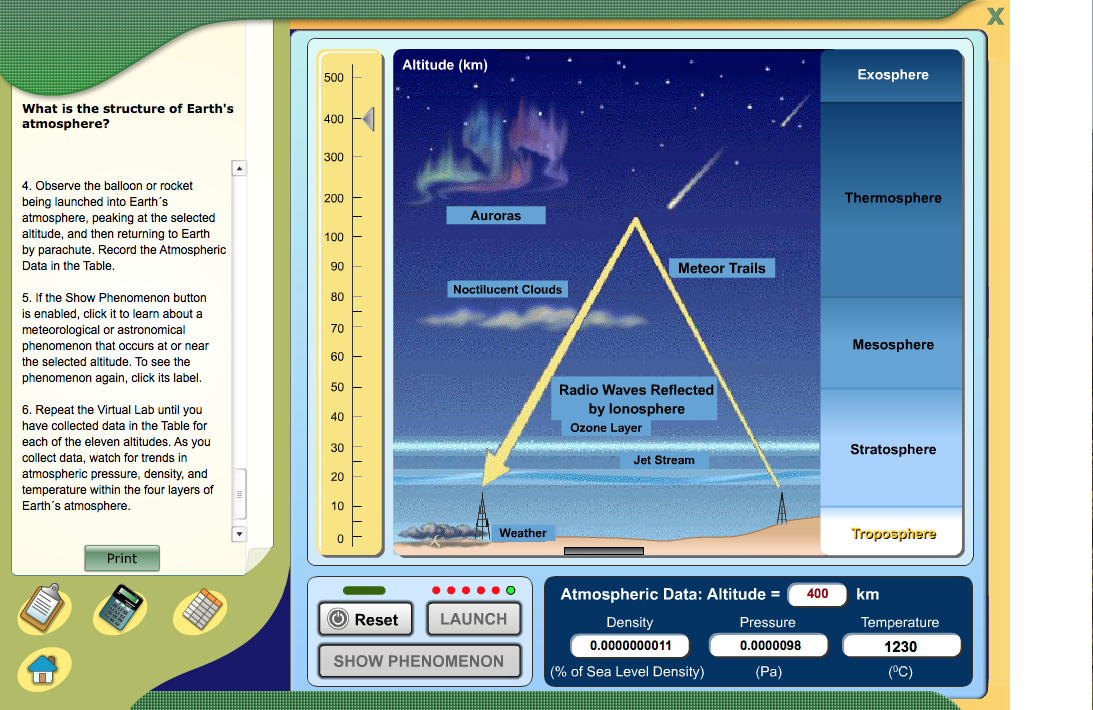This detailed colorized graphic appears to be a screenshot from an educational science program focused on the Earth's atmosphere. Dominating the center of the image is a diagram of the sky, featuring stars, auroras, noctilucent clouds, meteor trails, and radio waves reflecting off the ionosphere. The diagram is bordered by a vertical altitude scale, illustrating various atmospheric layers labeled from the troposphere up to the exosphere.

To the left, the graphic contains text headed by the question, "What is the structure of Earth's atmosphere?" This indicates that the image might be part of a lesson plan or test. The text includes instructions like "observe the balloon or rocket being launched into Earth's atmosphere, peaking at the selected altitude and then returning to Earth by parachute," hinting at an interactive element where users record atmospheric data.

The user interface is sophisticated, with multiple buttons at the bottom labeled "reset," "launch," and "show phenomenon," which suggest interactive features to explore atmospheric phenomena. A variety of icons, including a clipboard, calculator, grid pattern, and house logo, are situated on the lower left, implying additional functionalities or tools within the program.

Adding to the digital nature of this educational tool, there's a print button, salient white scroll bar, and the familiar small 'X' on the upper right-hand corner typical of a web browser or computer program. This alludes to an engaging, multimedia approach to learning about atmospheric science, blending text, interactive buttons, and vivid, instructive imagery.